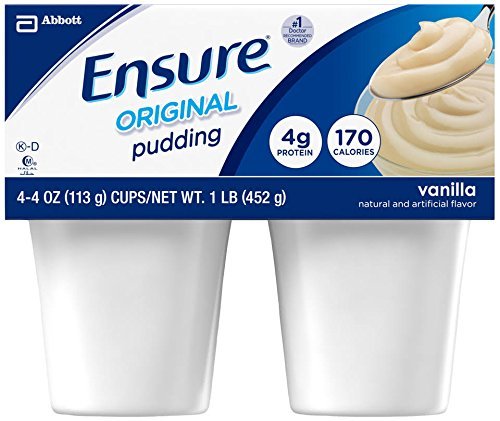This color photograph features a computer-generated image of a four-pack of Ensure Original Pudding in vanilla flavor. The packaging is primarily blue and white, adorned with the Abbott logo—a backward "A"—in the top left corner. The label prominently displays "Ensure Original Pudding" in blue letters with a gray circle nearby, noting it as the "Number One Doctor Recommended Brand." 

The package includes four four-ounce cups totaling a net weight of one pound. The product provides 4 grams of protein and 170 calories per serving. Additionally, there is an image of a bowl of yellow pudding with a spoon lifting a dollop of pudding above it. The two visible pudding cups are white and slightly flared, nested under the rectangular cardboard label that features swooshes of medium and dark blue along with white accents. The bottom blue band of the packaging indicates the flavor as "vanilla," naturally and artificially flavored.